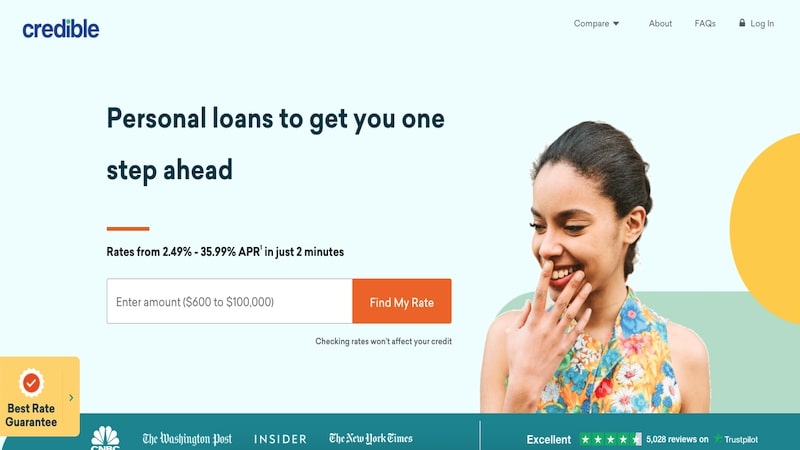This image features a well-organized and informative landing page for a financial service. In the top left corner, the word "credible" is prominently displayed in dark blue text on a light blue background. Positioned in the top right corner is a drop-down menu labeled "Compare," along with tabs for "About" and "FAQ." Additionally, there is a lock icon indicating a secure area for users to log in.

Dominating the center of the layout is a bold black headline reading, "Personal loan to get you one step ahead." Directly beneath this headline is a slender horizontal orange line, followed by a subheading stating, "Rates from 2.49% to 35.99% APR in just two minutes."

Below the subheading is an interactive search box inviting users to "Enter amount 600 to 100,000," accompanied by a vibrant orange button labeled "Find My Rate." A reassuring message is placed under the search box, promising that "Checking rates won't affect your credit."

To the right, the image features a woman dressed in a blue floral dress, adding a personal touch to the page. The bottom section of the image is framed by a light blue border, and includes logos from reputable publications such as CNBC, The Washington Post, Insider, and The New York Times.